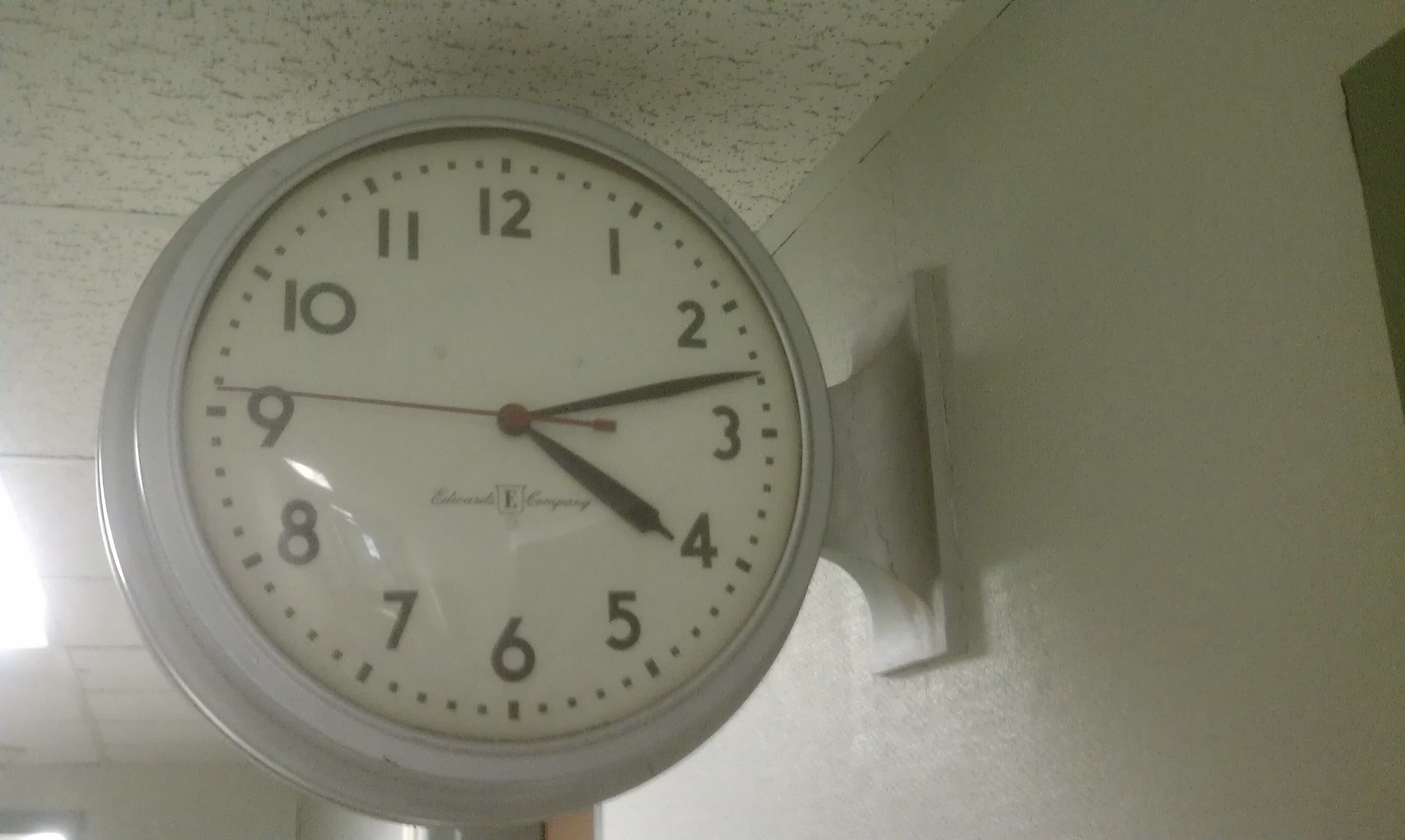A photograph showcases a minimalist, white circular clock mounted on a pristine white wall within a room or hallway. The impeccably clean background, painted in white, creates a cohesive look that blends seamlessly with the equally white ceiling. This standard, non-digital clock features a classic face adorned with bold black numbers from 12 to 11, organized in a clockwise fashion. The timepiece is equipped with three distinct black hands: a short, rectangular one for the hour, a longer rectangular one for the minute, and a thin, slender line for the seconds. The clock precisely displays the time as 4:13 and 45 seconds. The entire setting is well-lit, emphasizing the clock's clear readability and its functional elegance.